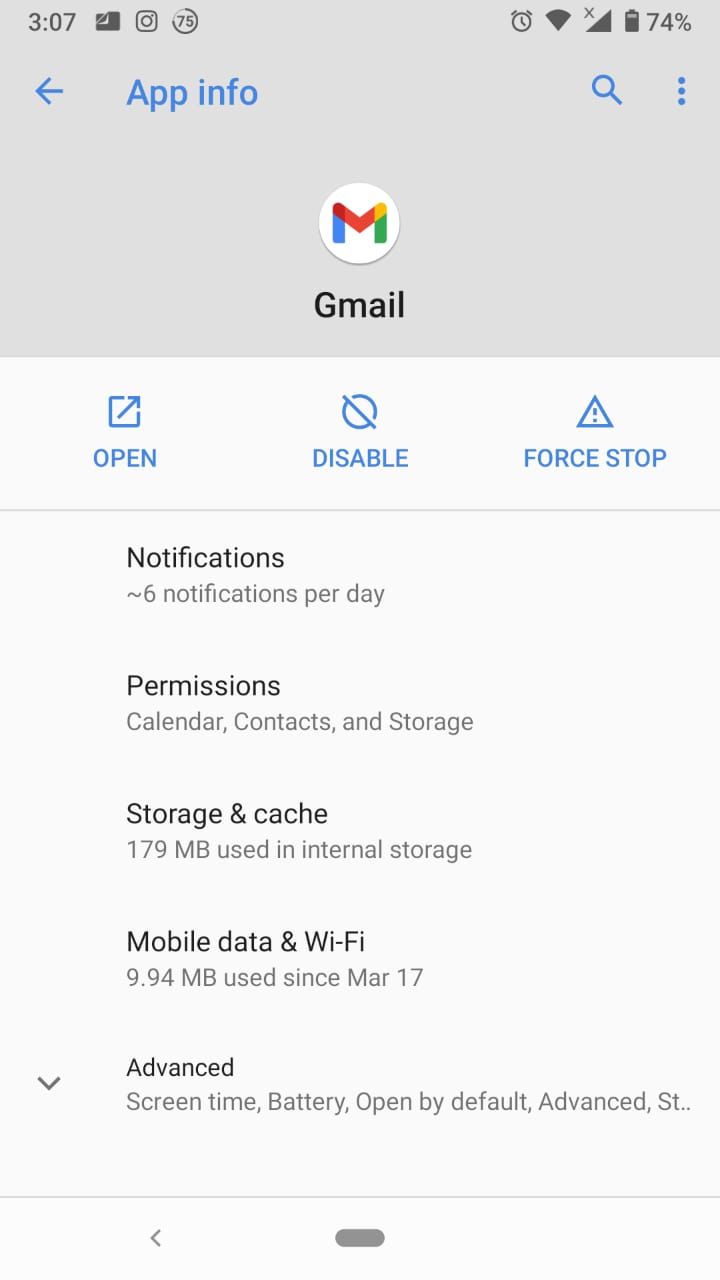The image shows a detailed overview of the Gmail app's settings screen on an Android device. 

In the upper left corner, the time is displayed as 3:07. Adjacent to it on the right is a vertically set black battery icon indicating a 74% charge. Just below this battery icon, a blue arrow points left, accompanied by the text "App info" in blue.

Centering the screen, a prominent white circle featuring a bold, thick-lined 'M' is displayed. This 'M' is designed using a combination of blue, red, yellow, and green colors, representing the Gmail logo. Beneath this, the word "Gmail" is clearly mentioned.

Further down, three interactive options are available: "Open," "Disable," and "Force stop." Notably, above "Force stop," a warning triangle with an exclamation point signals caution.

Continuing below these options, a long horizontal line separates the sections. Under "Notifications," it specifies "6 notifications per day" in black text. Following this, the "Permissions" section lists "Calendar, Contacts, and Storage."

Next is the "Storage and cache" section, noting that 179 MB is being used in internal storage. The "Mobile data and Wi-Fi" section states a usage of 9.94 MB since March 17th. Lastly, the "Advanced" section includes options for "Screen time, Battery, Open by default," and an additional "Advanced" subcategory.